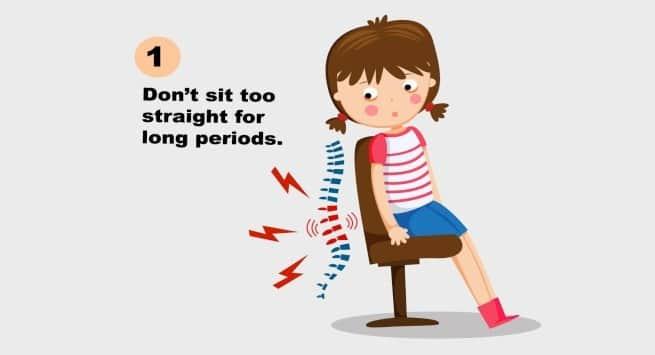The image is a horizontally long, rectangular infographic with a light gray background. At the heart of the design, slightly off-center to the right, is a cartoon depiction of a young girl with brown hair styled in pigtails. She is dressed in a white and pink striped t-shirt, a blue skirt, and pink socks, and she sits in a brown chair that appears to be fixed to the floor, facing right. Her face, adorned with ruby red cheeks and subtle pink circles under her eyes, is turned back to the left over her right shoulder.

Behind her is a detailed graphical representation of a spine, with the middle vertebrae colored red to illustrate stress or strain, while the sections above and below are blue. Cartoon lightning bolts and curved lines emanate from the red vertebrae, further emphasizing the discomfort caused by her sitting position. Beneath the chair is a gray circular shadow, grounding the image.

In the top left corner of the design, there is a small tan circle with a black numeral "1" inside it, which is followed by the black text: "Don't sit too straight for long periods." The entire scene is rendered in an educational style, with colors including gray, peach, black, red, blue, white, brown, and pink, giving it a straightforward yet engaging appearance suitable for an instructional guide or book.